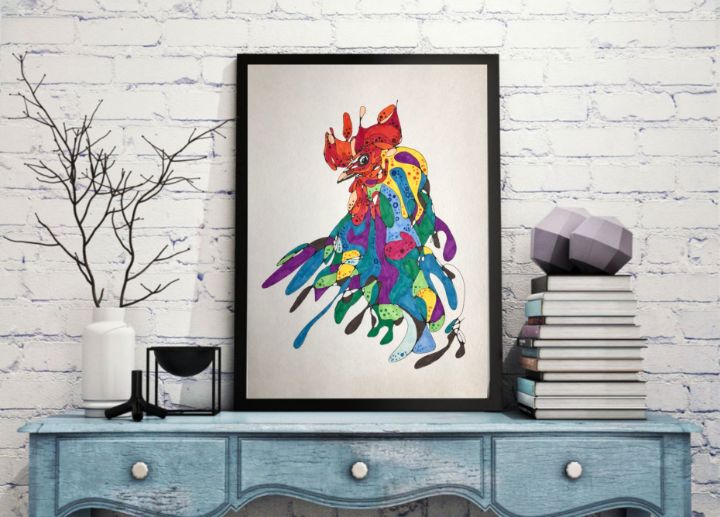The photograph depicts a charming, eclectic scene set against a white brick wall. At the center of the image is a distressed, blue-painted wooden desk with three drawers featuring wide, somewhat spiky handles. On the right side of the desk sits a neatly stacked pile of approximately a dozen books, topped with what appears to be a stylized drum.

Dominating the middle of the composition is a vibrantly colorful, framed picture of a rooster. The rooster, captured in a dance-like pose, is adorned with an array of multicolored feathers in shades of red, blue, yellow, purple, and green. Its head sports a quirky red cap instead of the usual comb, adding a whimsical touch. The picture is encased in a dark brown frame with a very slight beige inner border.

To the left of the image, resting on the desk, is a white vase that resembles a kettle. It contains a sparse arrangement of brown tree branches that extend upwards, contributing to the rustic feel. Another framed picture leans casually against the wall behind the vase, although its contents remain indiscernible. This stylistic tableau is both vivid and nostalgic, anchored by its blend of colors and textures, and the quirky rooster image serves as a lively focal point.